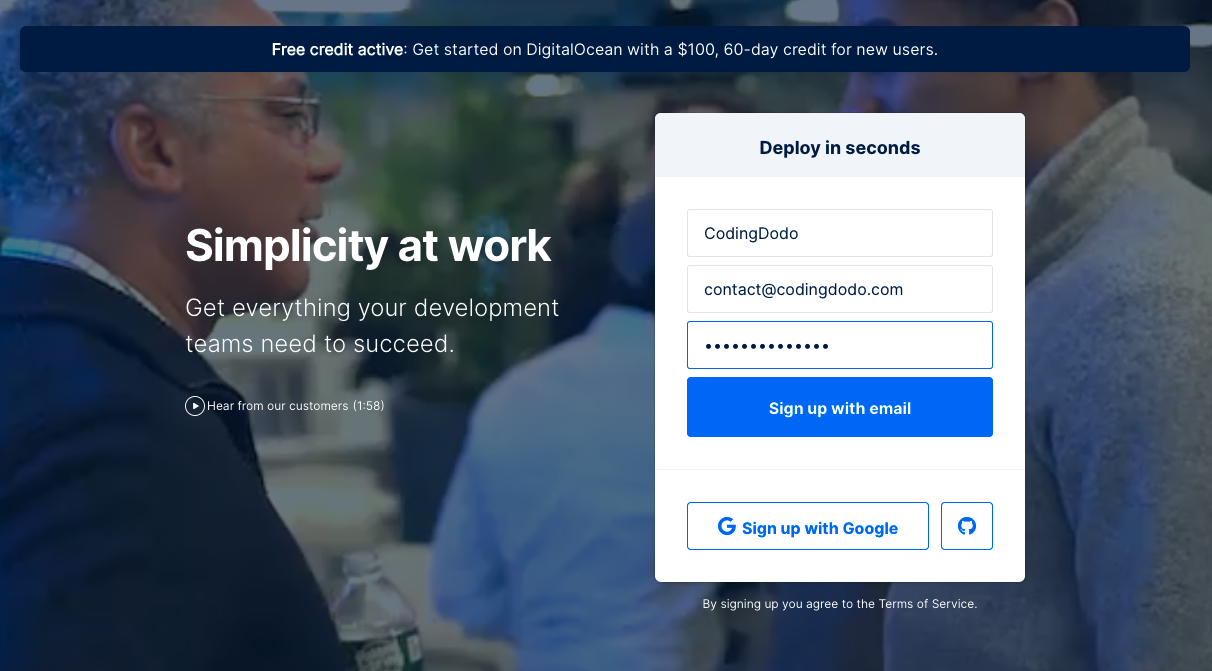**Caption:**

The homepage of the website features a dimly lit background photograph with a bluish tint, showcasing people mingling. On the left side of the image, a man wearing a blue suit jacket, with short gray hair and glasses, holds a clear water bottle and faces a man on the right dressed in a gray sweater with short brown hair. The background includes additional mingling people and a large potted plant in a blue vase.

Overlaying the background is a blue rectangle with rounded corners at the top. Centered within the rectangle is bold white text stating, "Free Active Credit:" followed by non-bolded text that reads, "Get started on DigitalOcean with $100 60-day credit for new users."

On the left side of the photograph, large white text declares "Simplicity at Work." Below this, two lines of smaller white text say, "Get everything your development team needs to succeed." Further down, there's an even smaller line of text accompanied by a white circle with a triangle inside it, next to the text, "Hear from our customers (1:58)."

On the right-hand side of the frame is a vertical white rectangle with rounded corners. The header at the top has a light gray background and bolded blue text that reads, "Deploy in Seconds." Against the white background are three text boxes: the top two with light gray outlines and the bottom one with blue outlines. The first text box contains the black text, "coding dodo," the second one reads, "contact@codingdodo.com," and the third one is filled with black dots. Beneath these text boxes is a button matching their shape, filled with blue, and features white text that says, "Sign up with email."